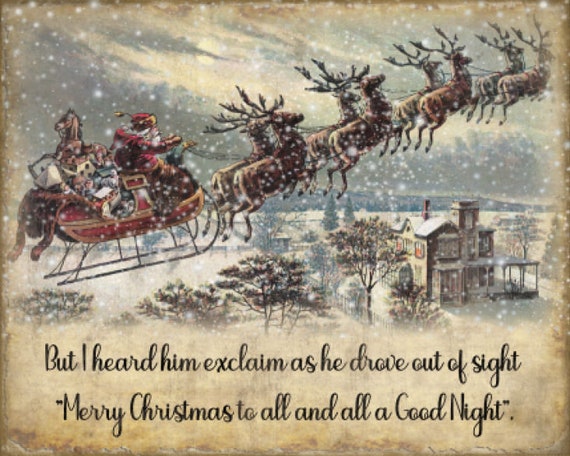This captivating painting showcases a classic Christmas scene of Santa Claus in his red and golden sleigh, overflowing with gifts such as a rocking horse and various other toys. Santa is being pulled by eight brown reindeer, arranged in pairs, as they soar diagonally across the snowy night sky. Below them, a serene winter landscape is depicted, featuring a neighborhood house surrounded by several snow-covered trees. The entire scene is set against a backdrop of a moonlit sky filled with snowflakes. At the bottom of the painting, a festive quote in cursive reads, "But I heard him exclaim as he drove out of sight, Merry Christmas to all and to all a good night." The painting is framed in a style reminiscent of old storybooks, with dark and rustic shades enhancing its nostalgic charm.